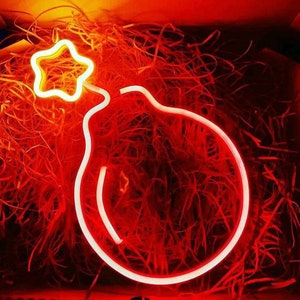The image features a vibrant neon sign shaped like a lightbulb with a five-pointed star extending outward from where the filament would typically be. The neon glows in hues of pink, red, and orange, creating a dynamic and colorful display. The lightbulb element includes a white line to symbolize a glare. Surrounding the neon sign, the background consists of intricate, intertwined red strands resembling thinly shredded paper or fibers, evoking a texture similar to red yarn or hay. The backdrop further consists of blackness, which enhances the vividness of the neon colors. Additionally, a bright orange light is noticeable in the upper left corner, adding to the image's overall luminous quality. There are no words or numbers present in the image, allowing the focus to remain on the striking neon light and its textured surroundings.